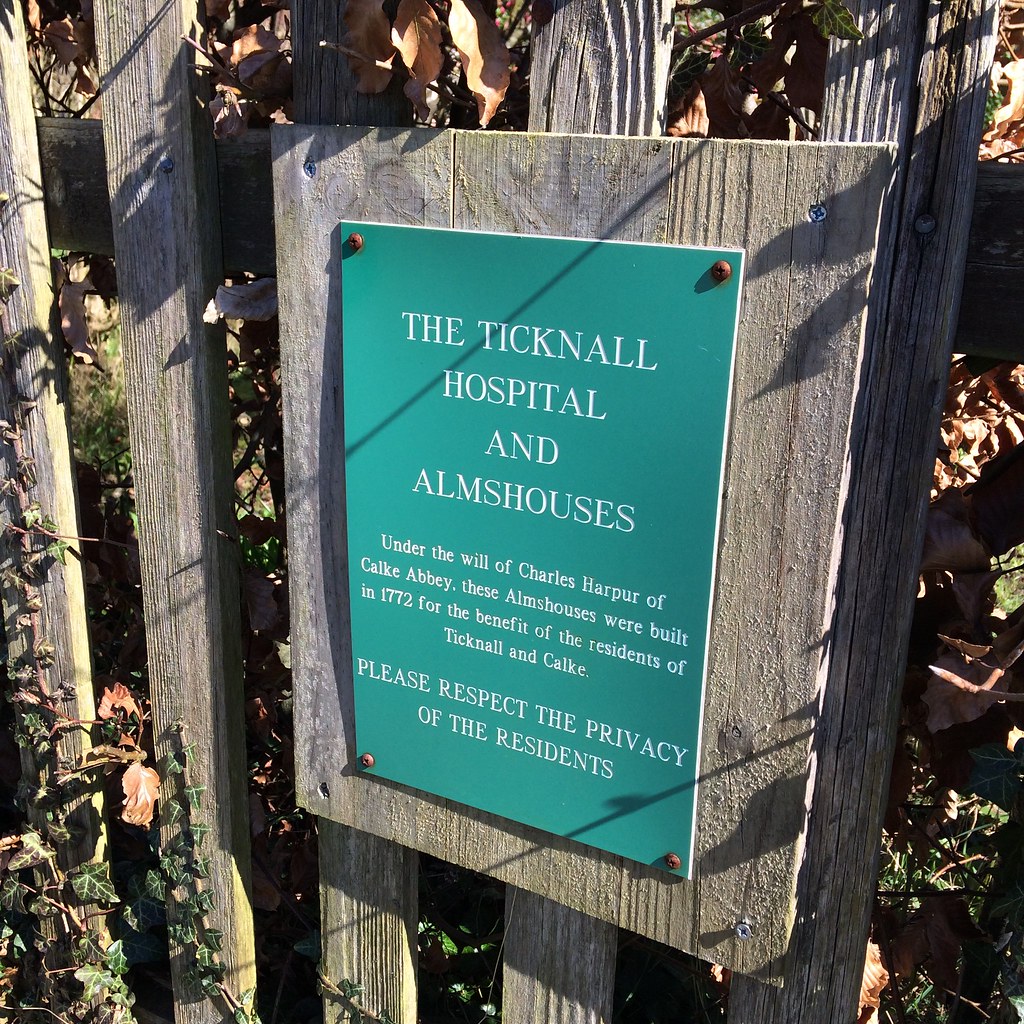This image displays a vertical, rectangular sign, affixed to a wooden plank fence. The fence is composed of vertically aligned strips of wood with small gaps between them. Behind and partially intertwined with the fence, lush green vines and some brown leaves are visible, embellishing the scene with natural elements.

The sign consists of a brown wooden backing, over which a solid green metal or turquoise blue plaque has been mounted. This plaque features white text and is slightly shorter and narrower than the wooden backing. The prominent heading on the plaque reads, "The Ticknall Hospital and Alms Houses," in larger white letters, emphasizing its importance. Below this, a paragraph in smaller white text states, "Under the will of Charles Harper of Calk Abbey, these alms houses were built in 1772 for the benefit of the residents of Ticknall and Calk." At the bottom, a respectful reminder in all capital letters asks, "Please respect the privacy of the residents."

The sign appears to serve both as a historical marker and a notice to visitors, informing them of the establishment's origin and purpose, while also requesting them to honor the privacy of the current residents.